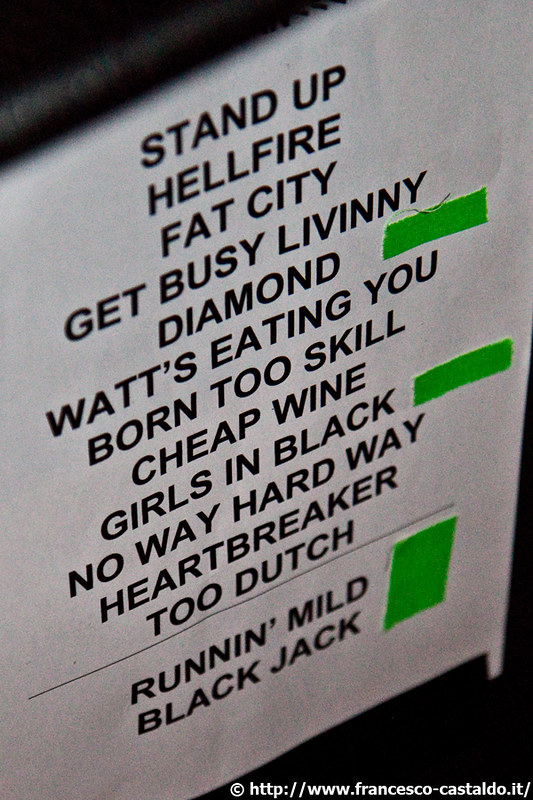This image captures a detailed close-up perspective of a white sign bearing a potential music band's set list, set against a stark black background, making the sign the focal point. The sign, possibly mounted on a window or wall, features bold black text listing song titles in order: Stand Up, Hellfire, Fat City, Get Busy, Liviny, Diamond, What's Eating You, Born to Skill, Cheap Wine, Girls in Black, No Way Hard Way, Heartbreaker, Too Dutch, followed by a black dividing line, and then Run and Mild, Blackjack. Adjacent to the words Diamond, Girls in Black, and the combined titles Run and Mild, Blackjack, there are pieces of green tape; the latter tape is notably larger and vertically oriented. The bottom-right corner of the sign includes a URL that reads "© www.francisco-castaldo.it," providing its copyright information.